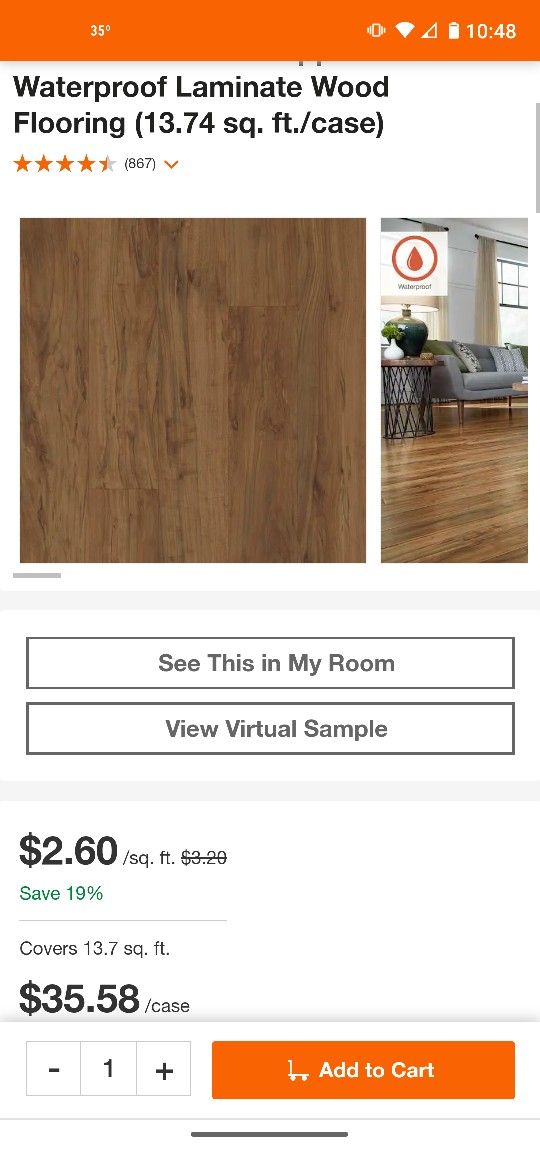A screenshot of a Home Depot website page showcasing waterproof laminate wood flooring. The orange Home Depot banner tops the page, displaying essential phone information such as the time (10:48) and an almost full battery, along with other status symbols. Beneath the banner, the page features a white background with bold black text reading "Waterproof Laminate Wood Flooring (13.74 sq. ft. per case)." The product boasts a rating of four and a half stars from 867 reviews, and an orange downward-pointing arrow indicates the option to read the reviews.

An image of the flooring, displaying its wooden finish, prominently occupies the center. A scroll button at the bottom hints at more pictures, including a preview of the flooring used in a living room. Below the images, options to "See This in My Room" or to view a virtual sample are available.

The flooring is on sale for $2.60 per square foot, discounted from the original price of $3.20, highlighted by green text indicating a 19% savings. Each case covers 13.74 square feet, priced at $35.58. Options to select the quantity and add the product to the cart are provided, with the familiar orange "Add to Cart" button reflecting Home Depot's signature colors.